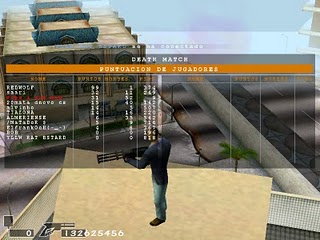This is a detailed screenshot from a video game displaying a Deathmatch scoreboard with white gamer tags listing kills, deaths, and ratios. The background features a vivid scene where a character, shown from a side profile, is holding a long-barrel, machine gun-type rifle. He is dressed in a navy blue shirt and aqua or blue pants. The character stands on what appears to be the roof of a building, with another building visible off in the distance, along with a grey roadway below. The sky behind him is clear and blue. Notably, you can spot a single palm tree amidst the mechanical, metallic imagery. Additionally, there are score boxes at the bottom left of the screen, one showing '0' and another displaying a string of seven numbers. The scene captures a third-person shooter perspective, emphasizing the character's readiness to engage in combat.